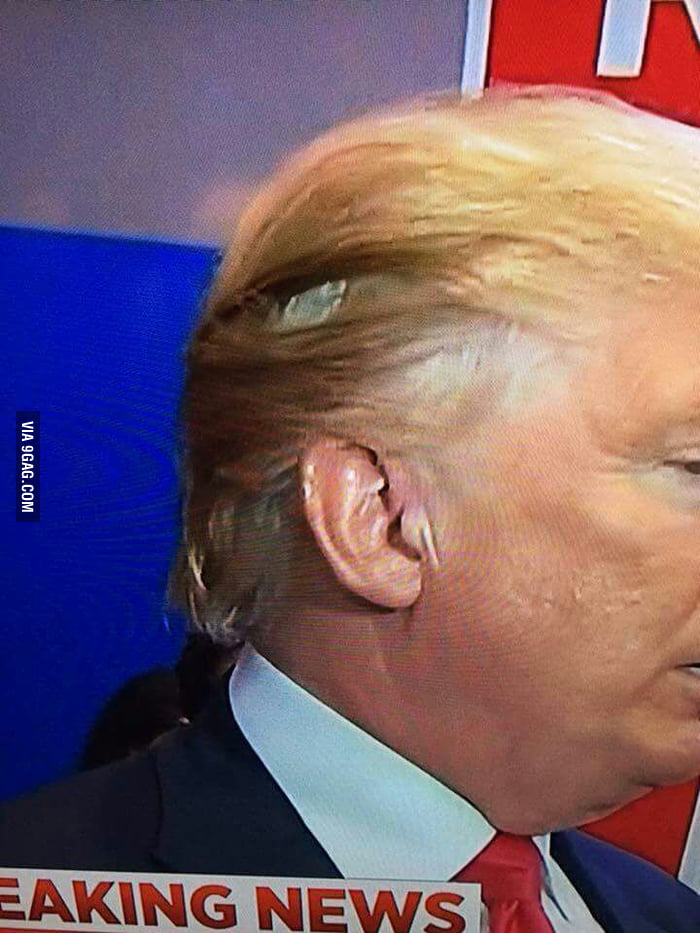This color photograph appears to be a fabricated still shot from a news broadcast, with the website “9gag.com” prominently displayed in the middle-left. The image features an up-close view of the right side of Donald Trump's face. His distinctive golden blonde hair is brushed back, partially revealing his ear, and he is dressed formally in a white shirt with a red tie and a blue jacket. The image's main focus is on Trump's hair, where an artificial-looking computer chip or implant is inserted, suggesting digital manipulation. At the photo's bottom, a ticker with the text “breaking news” is slightly misaligned, displaying as “eating news” instead. This, along with the "9gag.com" watermark, clearly indicates that the photograph is not authentic and has been digitally altered.